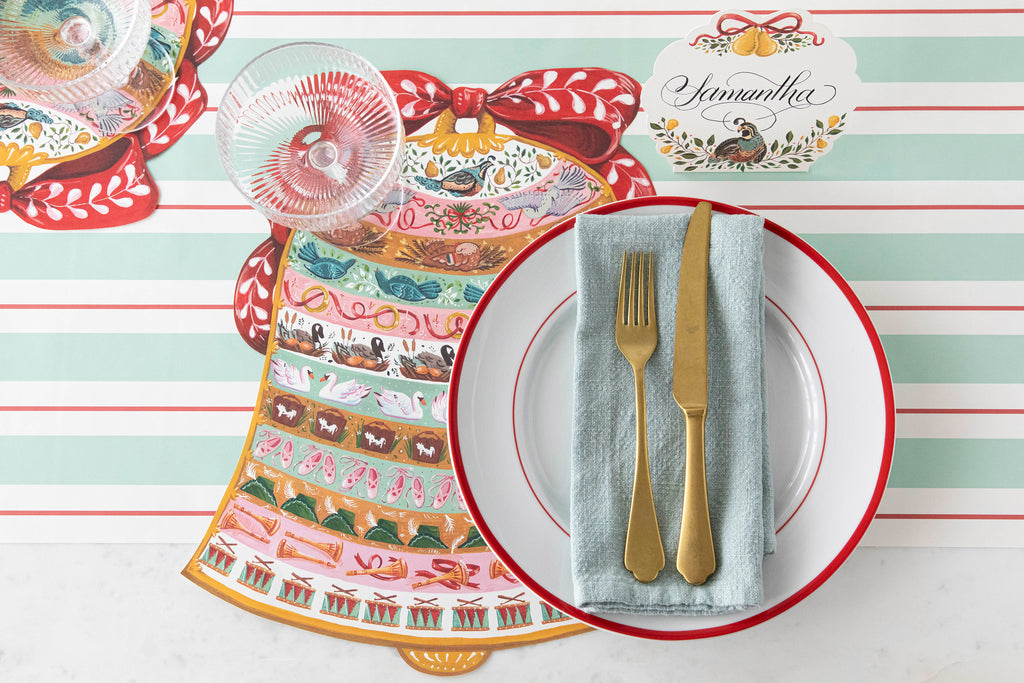This image depicts a festive place setting arranged on a table, evocative of a Christmas dinner scene. At the center is a white plate, adorned with a double red rim—a broad outer ring and a slender inner one. Resting on the plate is a linen napkin in a whitish-blue hue, paired with tarnished silver or gold-hued fork and knife. The plate is positioned on a vibrant placemat designed in the shape of a Christmas bell, featuring an intricate tapestry of seasonal motifs such as packages, trumpets, shoes, and swans. A red ribbon with white leaves delicately ties the bell design, enhancing the festive charm. To the top of the bell-shaped placemat stands an empty clear glass, likely intended for wine or another beverage.

Positioned to the right is a standout element—a crockpot-like design labeled "Samantha," adorned with two orange bells tied with a ribbon, and a rooster illustration with accompanying flowers below the name. Additionally, there's another place setting to the left, mirroring the arrangement with another empty glass. The overall color palette is rich and varied, featuring red, white, mint green, pale orange, brown, blue-green, and a goldish tone, all contributing to the image's vibrant and celebratory aesthetic.